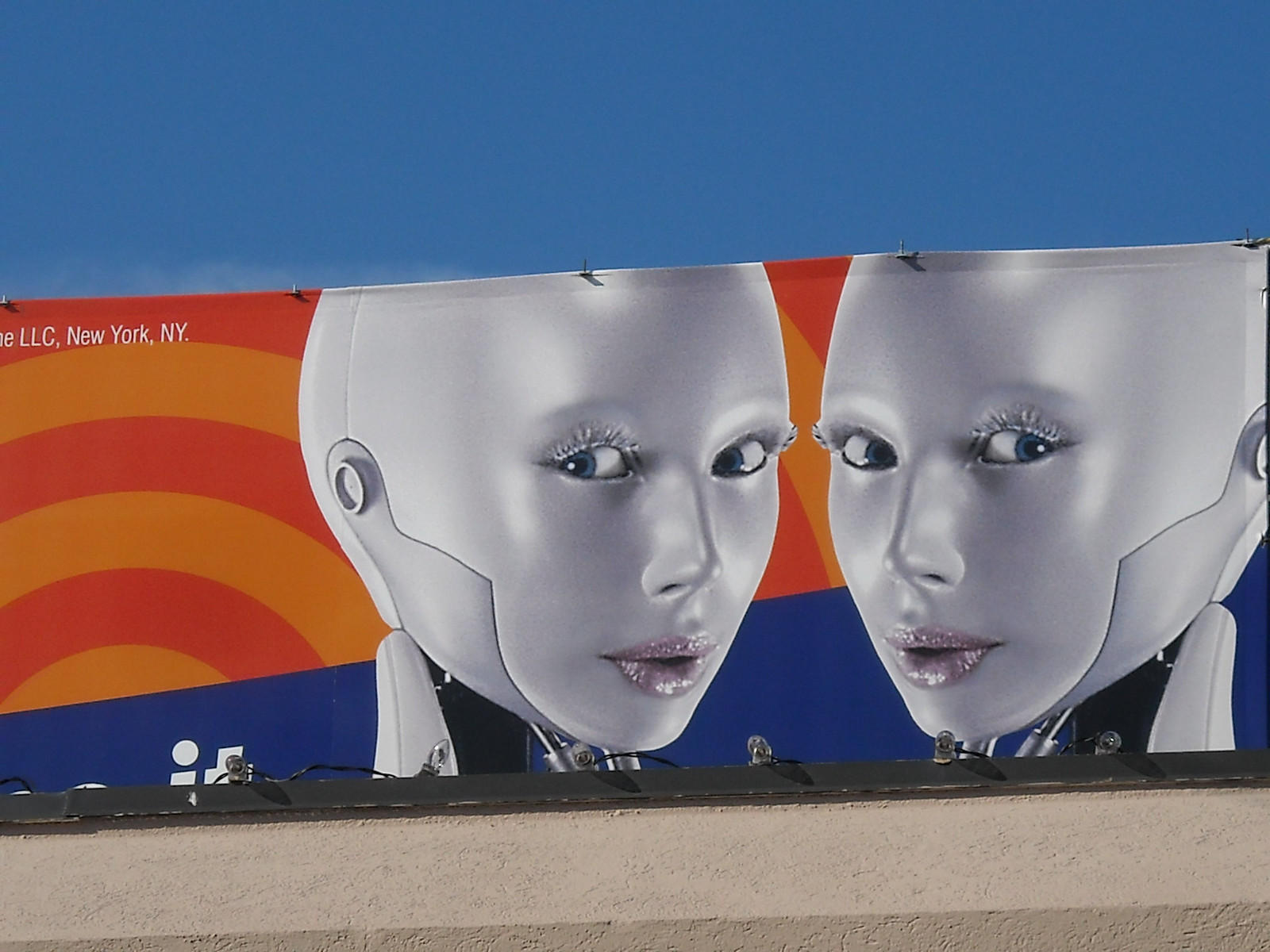The image depicts a large billboard situated atop a beige-colored building. Below the billboard, the building's concrete structure is visible. The focal point of the billboard features two white robots, positioned towards the right-center of the image. These robots are facing each other, but their blue eyes are directed towards the viewer. 

The robots' faces are detailed with glossy lips and have the appearance of being able to be disassembled, as indicated by a notable button-like feature on their jaws. Their necks, also white, are partially visible, with some black areas beneath their chins.

The background of the billboard consists of a gradient blend of orange and blue hues. In the top left corner, there is text that reads "New York NY LLC." The sky above the scene is a clear, bluish color, providing a contrasting backdrop for the futuristic visuals on the billboard.